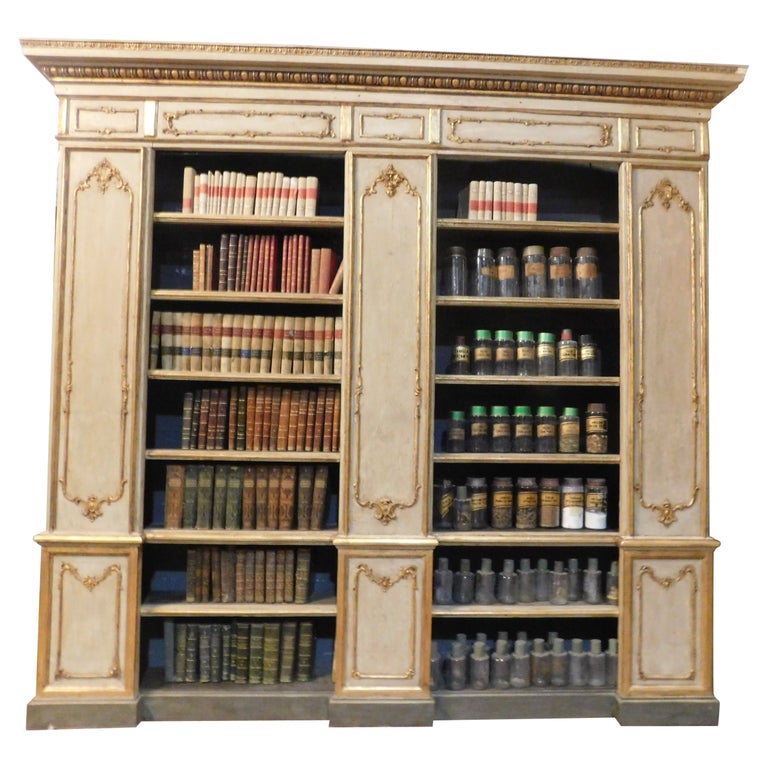This photograph depicts an ornate, classic bookshelf divided into two distinct sections, each comprising six shelves. The bookshelf features intricate thick wood paneling with gold decorations, crafted in an oval shape, which adorn the outer edges and the central pillar that separates the two sections. The shelves and the main structure are a tannish white color that matches the tan base at the bottom, complementing the lavish design.

On the left section, every shelf is filled with a collection of books, characterized by their consistent styling, hinting at series or sets of books meticulously organized with bookends. In contrast, the right section has a solitary top shelf occupied by books, while the remaining shelves display various glass jars, all featuring tan labels and containing different substances like powders and possibly dried leaves. Some jars appear aged and dusty, adding to the rustic charm of the piece.

Crowning the top edge of the bookshelf is elegant molding, which, along with the repeated gold ornate flourishes at the top and bottom of each inner frame within the three vertical columns, amplifies the overall elaborate and classic aesthetic of the bookshelf against its completely white background.